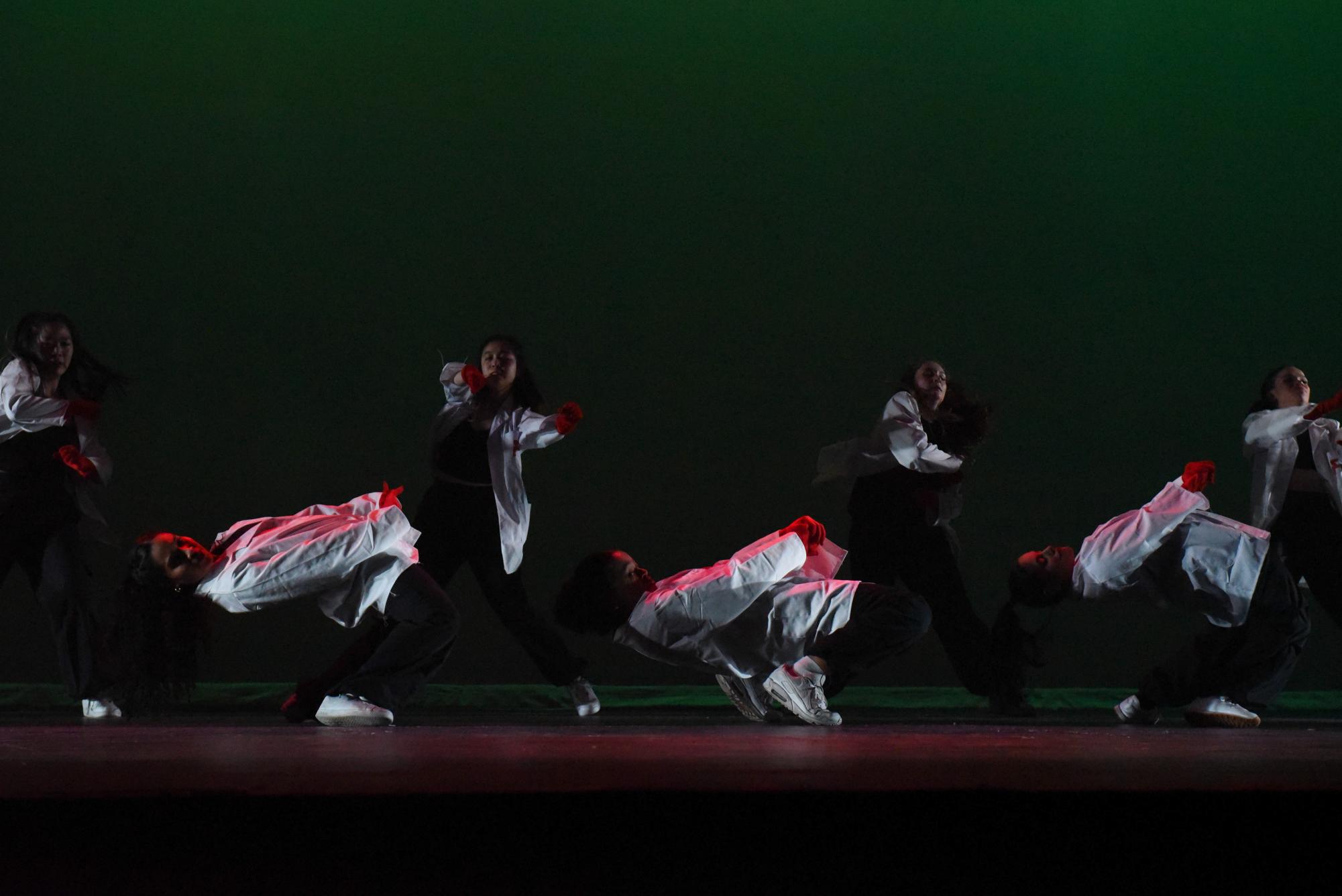The image captures a dynamic dance performance on a stage featuring seven female dancers, each clad in a coordinated costume consisting of a white button-down shirt, a black tank top underneath, black pants, white sneakers, and bright red gloves. The stage is dramatically lit, with vivid green lighting illuminating a solid scrim or curtain backdrop, and intense red light bathing the dancers from the front, creating a high-contrast, vibrant scene. Four dancers in the background are energetically moving their arms with feet planted wide, while the three dancers in the foreground are dramatically arching their backs towards the floor, their bodies almost parallel to the stage. The photograph, likely taken with a digital camera, captures the live energy and striking visual effects of the performance.